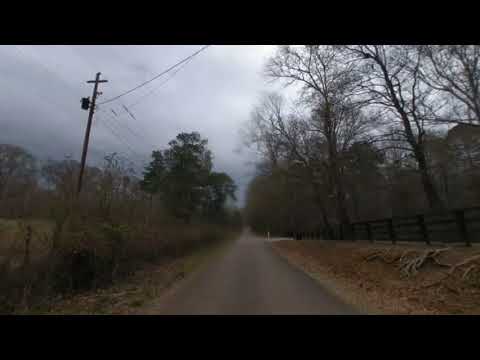The image captures a dreary, overcast scene on a rural country road, suggesting it may have recently rained. Central to the composition is a dark gray, narrow road, likely a one-lane path, flanked by patches of dirt, grass, and light-brown shrubbery. The road is unmarked and appears wide enough for one to two cars. To the right of the road, an embankment rises, featuring exposed roots and surmounted by a dark brown wooden fence with three horizontal planks between vertical posts. Behind the fence, taller trees create a dense background. On the left side, a thin line of smaller bushes and trees transitions into an open field visible in the distance, with light brown shrubbery partially obscuring an old wooden fence. A power line pole stands beside the road, with wires stretching toward the top right of the image. The sky above is a dull gray, contributing to the scene's overall somber tone. In the distance, about halfway down the road, there's a turning point where another path veers off to the right, adding depth to the rural landscape.